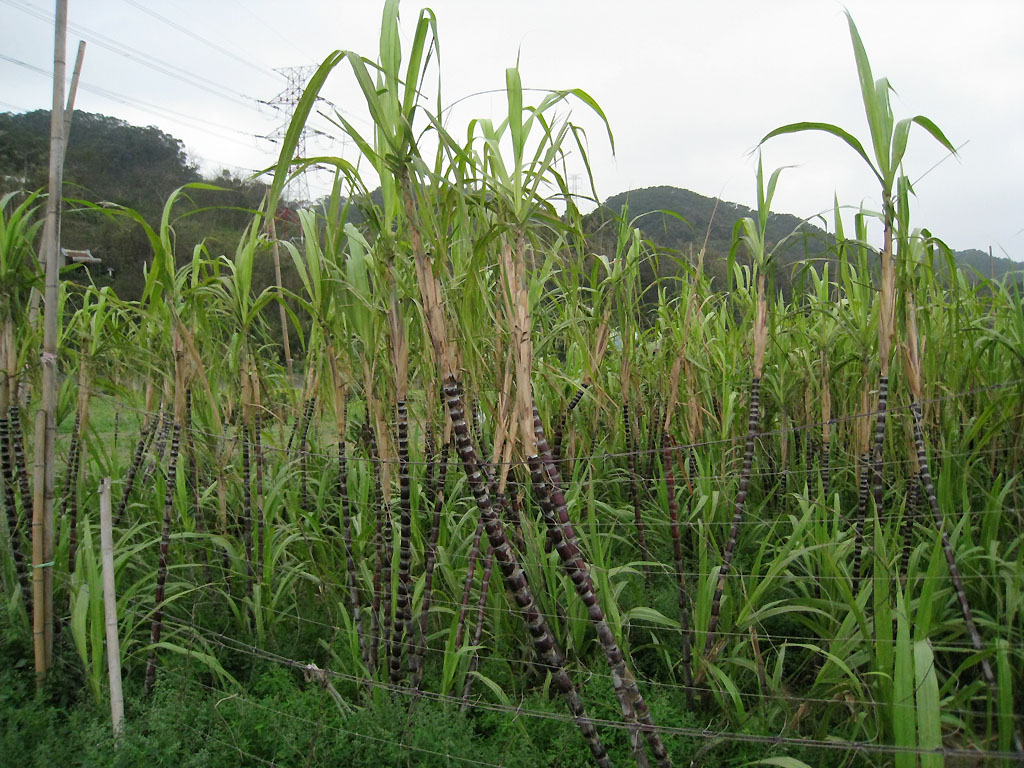The image showcases a lush tropical landscape dominated by a cloudy gray sky, which sets a somber and overcast mood. In the foreground, there is a metal mesh fence combined with an electric wire fence, creating a secure enclosure. Behind this barrier, there is a dense growth of distinctive plants, likely some type of cane plant with segmented brown stalks and narrow blade-like green leaves hanging from the top. Among these plants, there appears to be a short and a long bamboo reed tied together with a string, alongside a white piece of PVC pipe lying outside the fence. The background features an expanse of verdant hills and small mountains, blanketed in thick forest. Adding to the rural setting, an electricity pylon stands prominently with its cables stretching out across the landscape, disappearing into the distant, misty horizon.